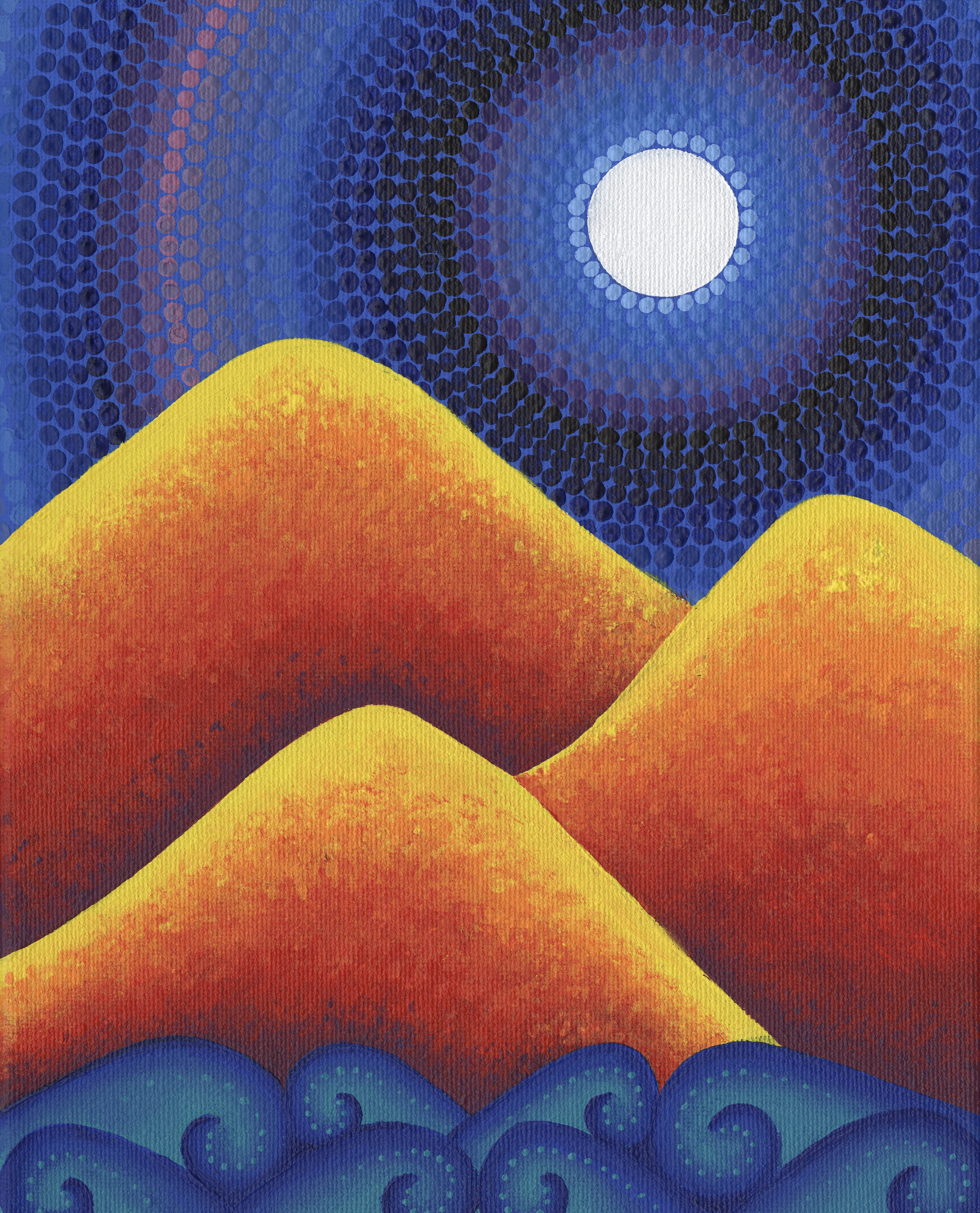The image is an unusual and abstract illustration featuring an ocean, three mountains, and a night sky. The ocean is depicted with large, oval shapes in a gradient of blues, from light to dark, and is accented with little dots to suggest waves. Above the ocean, three simplified mountains are arranged: the smallest mountain in the front, a medium-sized mountain to the right behind the smallest, and the largest positioned at the back. The mountains display a striking gradient that transitions from dark red at the base to orange and yellow at the peaks, echoing a vibrant sunset or lava-like appearance. 

The sky behind the mountains is crafted using a dot painting technique. At the center, slightly to the right, is a full, white circular moon. Surrounding the moon are concentric rings of dots that radiate outwards, changing colors from light blue to dark blue, purple, black, and eventually pink before repeating. These dots create a cosmic, starry night effect that contrasts beautifully with the vibrant, fiery mountains and the serene, wavy ocean below. The entire scene is highly illustrative, offering a visually rich and textured representation of a surreal landscape.